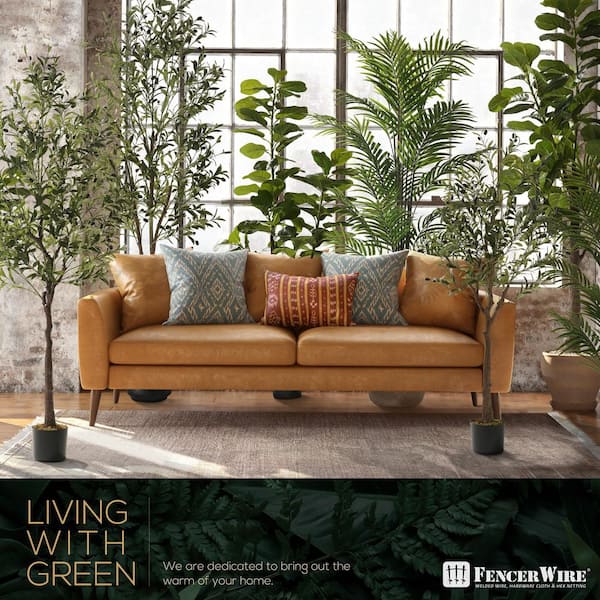The image depicts an indoor room lushly decorated with an array of verdant plants, including palm trees and other types of greenery, all neatly potted. The space is warmly illuminated by a large window with multiple panes and trim lining the wall behind the plants. At least six tall greenery pots are strategically placed to create a natural, indoor garden ambiance. Central to the room is a modern, light brown leather couch adorned with a variety of decorative pillows—some matching the couch's hue, while others introduce splashes of blue, white, and red with gold accents. In front of the couch lies a gray rug that features the text, "Living with green, we are dedicated to bringing out the warmth of your home." The rug is branded at the bottom with the name "Fencer Wire," signifying the company's commitment to enhancing indoor spaces with greenery. The overall setting showcases how integrating green plants can add warmth and vitality to home interiors.